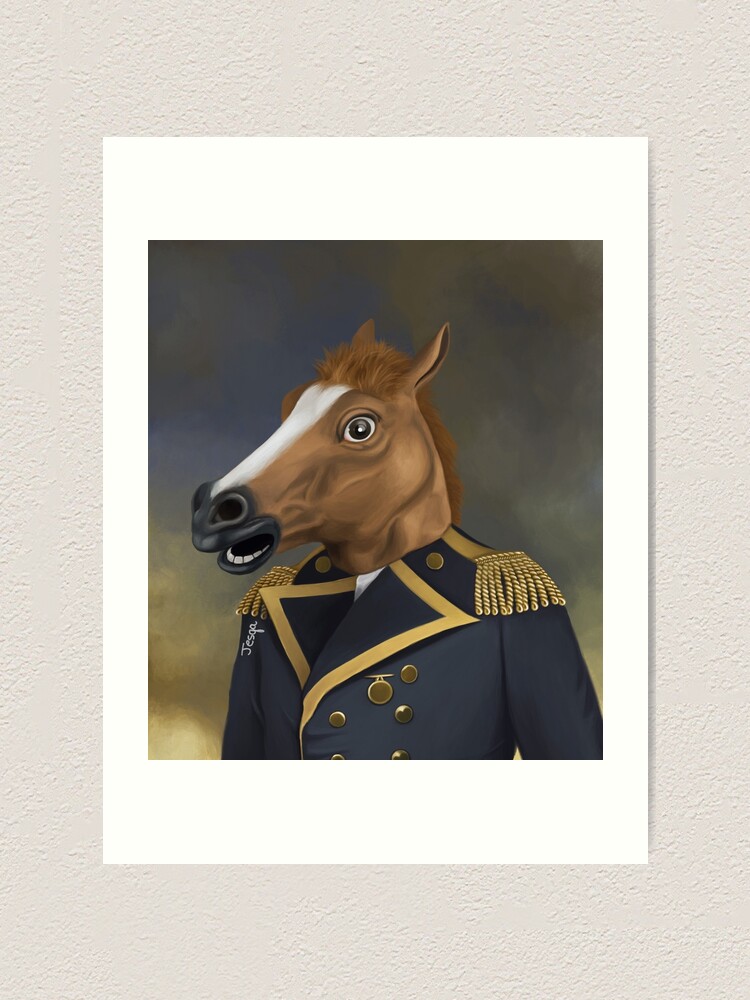This digitally rendered artwork features a whimsical and humorous portrait of a person with the head of a cartoonish brown horse. The horse, depicted in profile with its mouth open and a bewildered expression, has a distinct white stripe running down its face and is looking off to the side. The horse wears a navy blue admiral's military uniform adorned with gold accents, including a wide-collared lapel trimmed with gold, gold fringe epaulettes, and numerous gold buttons on the right side of the uniform. A medal is visible on the front sleeve, adding to the detailed rendering of the attire. The background of the image has a slight texture and is predominantly a greenish hue. The entire piece is printed on a poster with a thick white border and is hung on a textured beige wall. There is a signature along the left side of the poster, reading "Jessica," spelled as "J-E-S-Q-A," amidst the cloudy, abstract background.